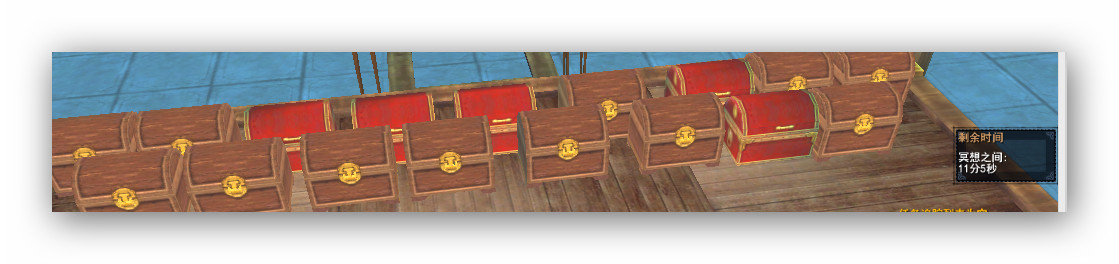The image is a color photograph in landscape orientation, depicting 17 traditional, treasure chest-like boxes neatly aligned on a light brown hardwood floor. The chests are organized in two rows, with the front row containing eight chests, among which seven are brown with light brown trims and circular emblems featuring a face on the front, and one is red with a gold trim. The back row includes nine chests, five of which are red with gold trims, while the remaining four are brown, also adorned with the same gold emblem. The chests, reminiscent of old-fashioned construction worker lunch pails, are sitting on a wooden platform that is placed on a blue or gray tile floor. Additionally, there's a small pop-up window on the right side displaying Chinese characters and numbers.